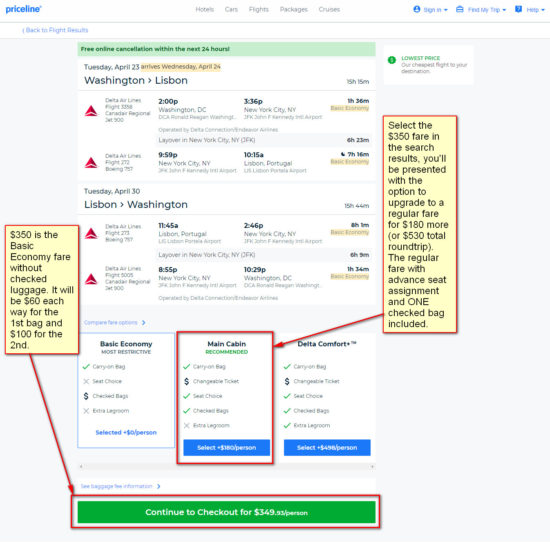Screenshot Description of Priceline Website:

The screenshot captures a detailed view of the Priceline website interface. 

1. **Header Area:**
   - **Top Left Corner:** The Priceline logo is prominently displayed.
   - **Top Middle Section:** A subtitle menu lists the available travel options: Hotels, Cars, Flights, Packages, and Cruises.
   - **Top Right Corner:** Three clickable options are visible, each with an accompanying arrow: Sign In, Find My Trip, and Help. 

2. **Navigation Breadcrumb:**
   - Beneath the header is a breadcrumb navigation link titled "Back to Flight Results."

3. **Notifications and Banners:**
   - Below the breadcrumb is a prominent green banner with the message "Free Online Cancellation within the next 24 hours."
   - Followed by a box highlighting "Lowest Price."

4. **Flight Information Overview:**
   - **Date**: Tuesday, April 23rd (Departure) and Wednesday, April 24th (Arrival).
   - **Locations**: Washington (Departure) to Lisbon (Arrival).
   - A comprehensive list of flight details is provided.

5. **Flight Schedule Details:**
   - **First Segment:** Takes off from Washington, D.C. at 2:00 PM, arriving in New York City at 3:36 PM (1-hour and 36-minute flight).
   - **Second Segment (Delta Flight):** Departs from New York City at 9:59 PM, arriving at 10:15 AM the next day (7-hour flight).
   - **Third Segment (Return Flight):** Leaves Lisbon at 11:45 AM, landing in Washington at 2:46 PM.
   - **Fourth Segment (Delta Flight):** Departs at 8:55 PM, arriving at 10:29 PM.

6. **Flight Options:**
   - Different fare classes are available: Basic Economy, Main Cabin, and Delta Comfort Main Cabin. 
   - The Main Cabin fare is recommended and highlighted.
   - Selection box available indicating "Select $350 Fare."
   - Additional upgrade options are mentioned: upgrading to regular fare for an additional $180, making it $530 total round trip. This fare includes advanced seat assignment and one checked bag.

7. **Call to Action:**
   - At the bottom of the screenshot is a prominent green button labeled "Continue to Checkout."